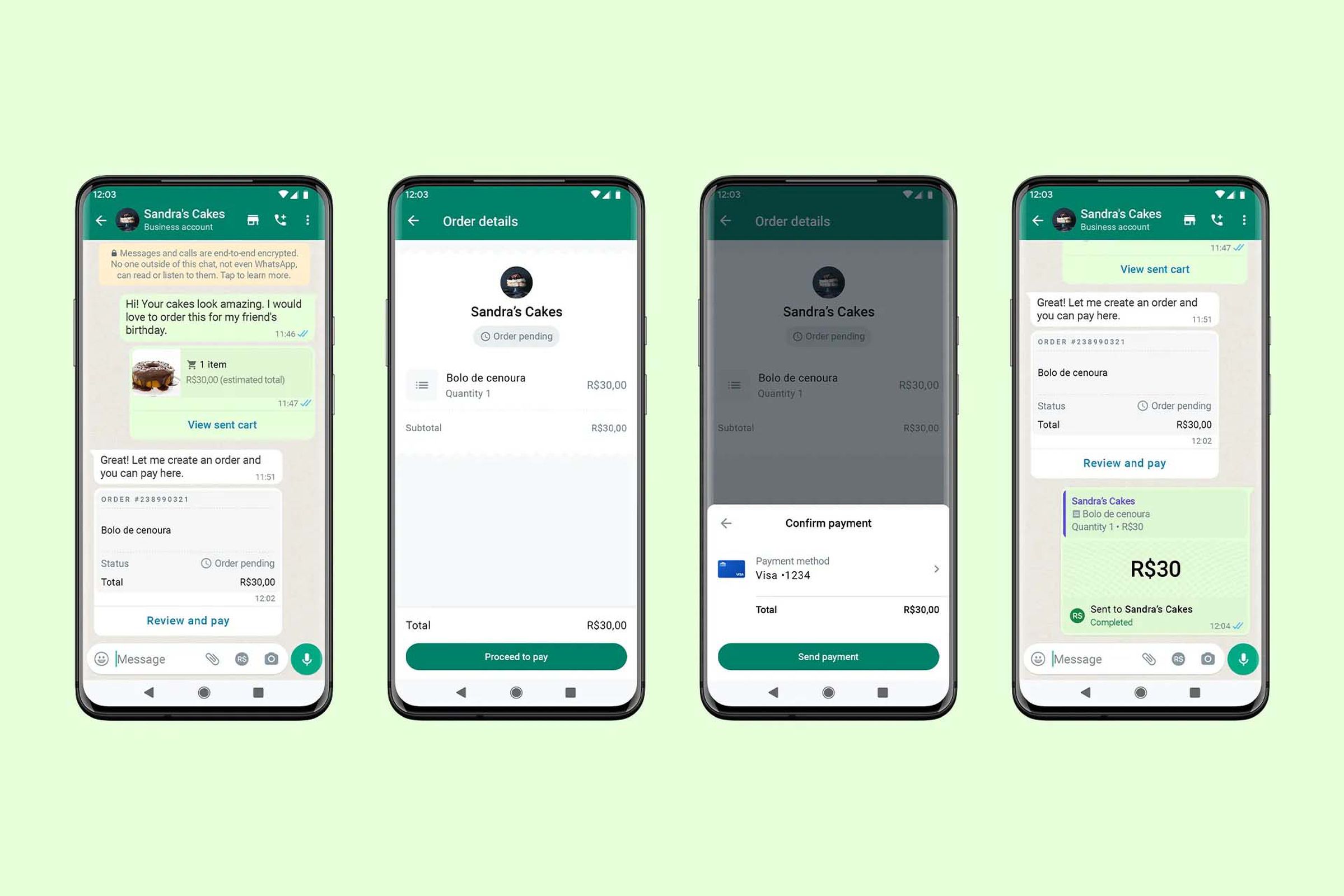This image is a detailed tutorial on how to send a payment through a specific web app, depicted on four iPhone screens against a light green background. 

1. **First Screen:** Shows a text message conversation with a contact named "Sandra Cakes," where a cake order is being placed. Sandra Cakes responds with the bill for the order.
  
2. **Second Screen:** Displays the detailed bill, which totals 30 units of a currency denoted by "R" followed by a dollar sign. A button labeled "Proceed to Pay" is visible for the user to continue the transaction.

3. **Third Screen:** Presents a payment interface where the user enters their Visa card number and confirms the total amount of payment, then clicks on a button labeled "Send Payment."

4. **Fourth Screen:** Returns to the text message interface, confirming that the payment of $30 has been successfully sent to Sandra Cakes.

The overall design features a simple and intuitive color scheme of green, gray, and off-white, making it easy to understand the payment process.